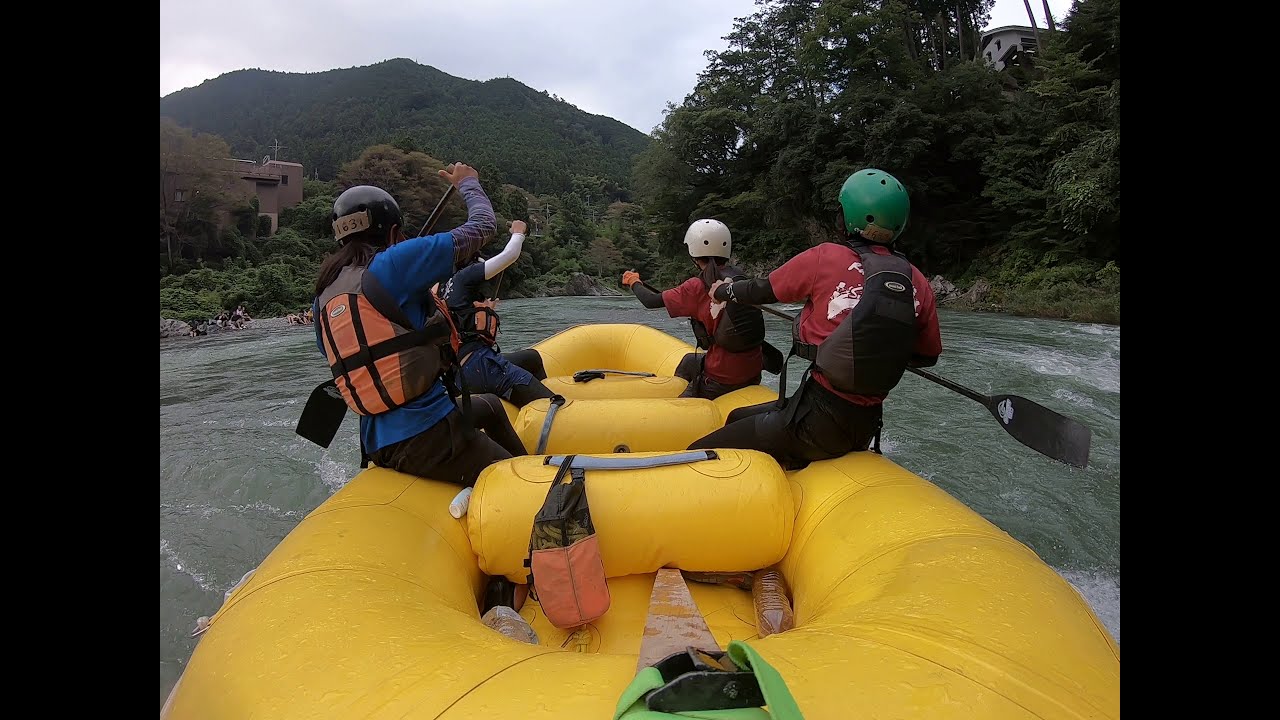A vibrant, detailed scene captures four individuals navigating a greenish-blue river in a bright yellow inflatable raft. All participants are equipped with life vests—two in orange and two in black. They sport various colored helmets: one green, one white, one black, and the last turquoise. Their outfits are diverse, with notable mentions including a red shirt with white writing, black pants, a dark blue T-shirt over a long-sleeved shirt, and an orange form-fitting backpack. Each rafter grips a paddle, some cutting through the water, others poised above it. A closer look reveals one person with a visible ponytail streaming from their white helmet, adorned with the number 1631. An orange bag containing rope hangs off the raft's seat.

The water flows with considerable movement, contrasting against the serene, overcast sky. Green hills densely covered with trees frame the background, punctuated by a white house perched on a hill and a brown brick building further downriver. Additionally, a gray concrete structure is visible on the left side near the center of the photo. The presence of people standing on the shore further enriches the scene.